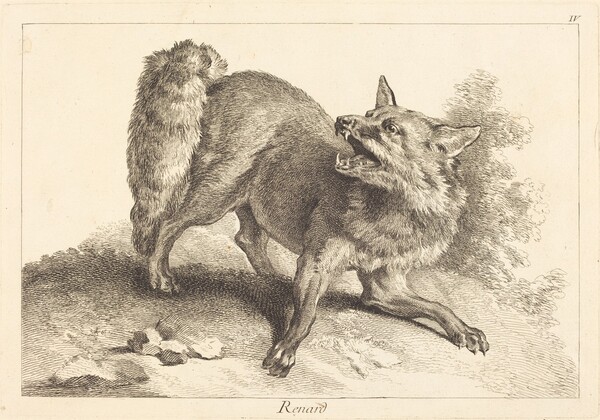The photograph showcases a detailed pencil drawing on cream-colored, rectangular A4 paper with a light pencil border. Dominating the center of the artwork is a naturalistic depiction of an animal resembling a wolf or a fox, identified with the French word "RENARD" inscribed at the bottom center. This creature stands on a small, stony ground patch, poised as if on a cliff, and is surrounded by some shadowy plant-like features. The animal's mouth is open, appearing to snarl or roar, with its head turned back towards its unusually wide, bushy tail located in the upper left. Its fur is meticulously sketched, emphasizing the texture and wild nature of the creature. The number "4" is faintly visible in the upper right corner of the drawing, adding a subtle detail to the composition.